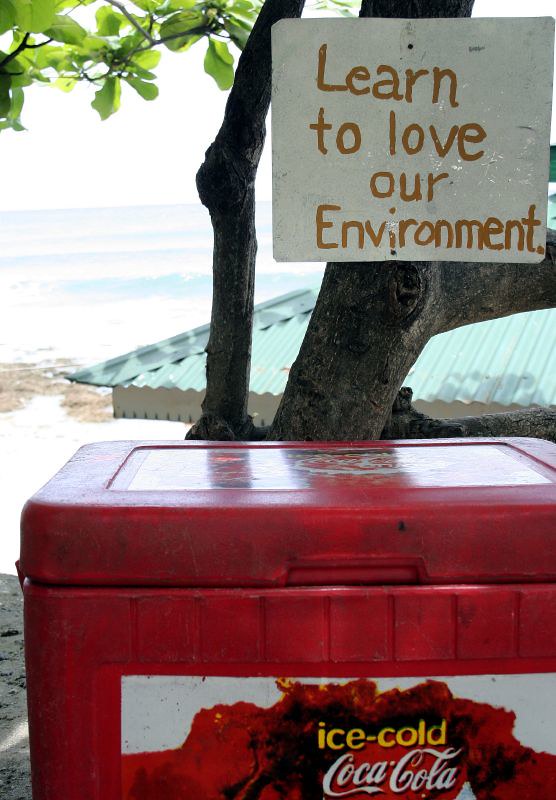The photograph depicts a well-used, red plastic Coca-Cola cooler prominently placed in the foreground, bearing a sticker that reads "Ice-Cold Coca-Cola" in classic white cursive lettering against a red background. The cooler itself appears quite beaten up, indicating it has seen a lot of use over the years. Behind the cooler is a tree with a handmade sign attached to its trunk. The sign is a white tin with brown, handwritten letters conveying the message, "Learn to love our environment."

In the background, beyond the tree, there is a pavilion or some form of building with a metal roof, likely indicating a picnic area. Further beyond the building, a sandy beach and a vast expanse of water, possibly an ocean, can be seen, suggesting that the scene takes place in a coastal area reminiscent of the Caribbean. Some green leaves are also visible in the upper left corner, adding to the scenic, natural setting. The overall scene appears to be one of a beachside gathering spot, highlighted by the iconic Coca-Cola cooler, the environmental message on the tree sign, and the serene coastal backdrop.